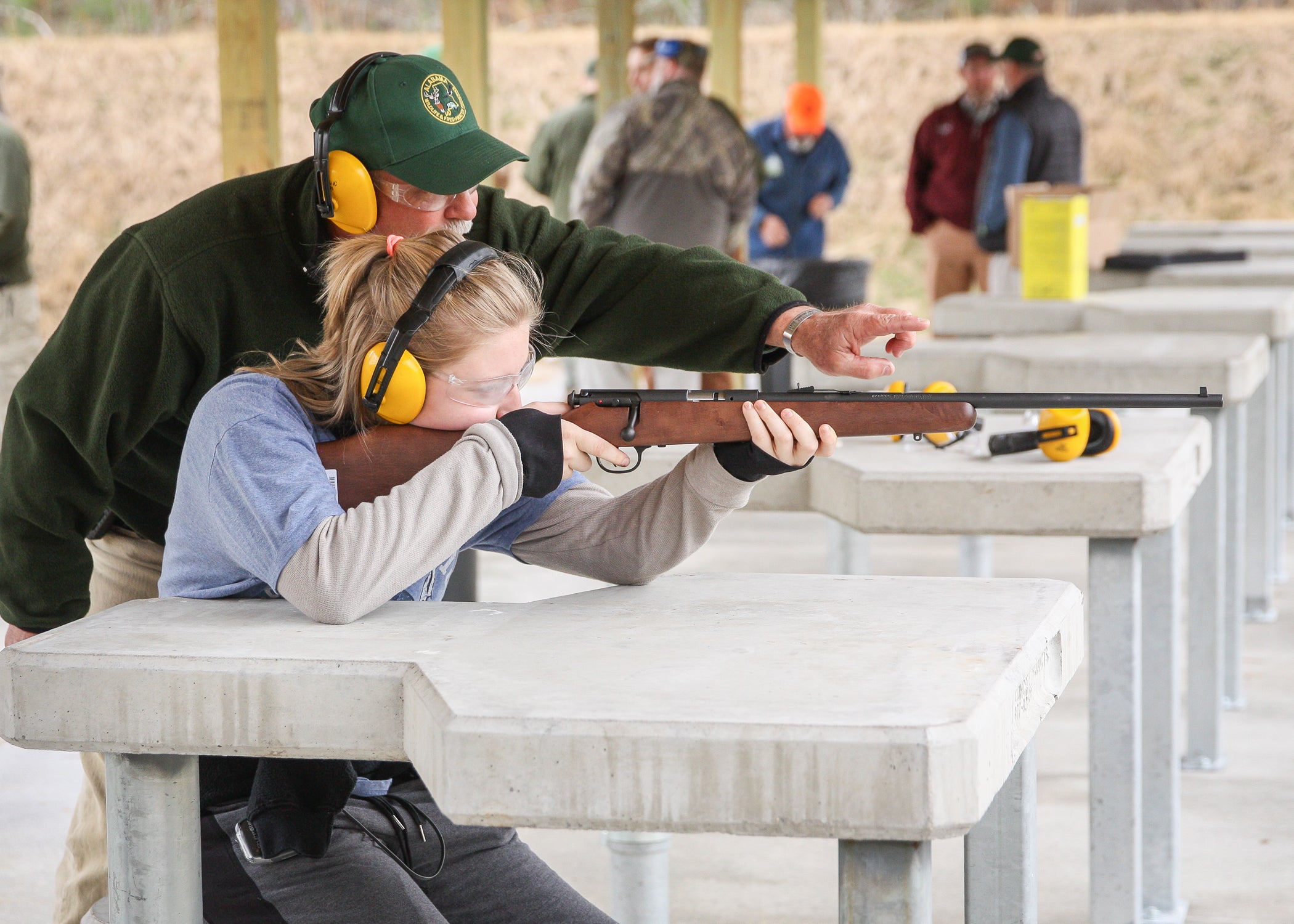In a bustling target shooting range with several concrete tables, the photograph captures a young teenage girl seated at the closest table in the foreground. Dressed in black pants, a blue t-shirt over a long gray sleeve, and equipped with yellow ear protection and safety glasses, she intently focuses on her rifle. Her elbows rest on the table as she aims towards the right of the frame. Crouched behind her, offering guidance, is a middle-aged man who appears to be of grandfatherly age. He wears a dark green jacket, matching green hat, tan pants, yellow earmuffs, safety glasses, and a silver bracelet. His mustache is visible as he points to the right, instructing the girl on better aim. In the background, more concrete tables and onlookers can be seen, adding to the active atmosphere of the shooting range.